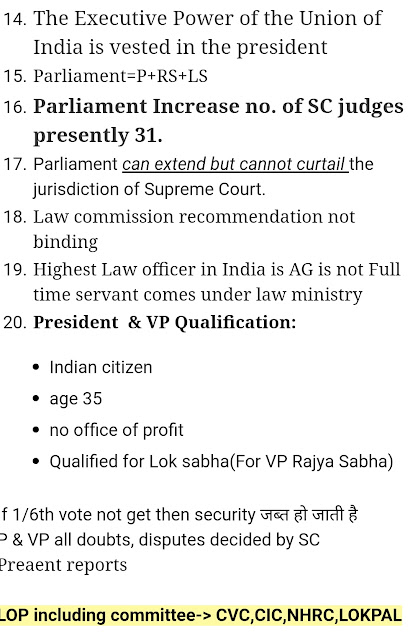This image appears to capture a fragment of a website featuring legal and political information related to India. At the top left corner, the image starts with the number "14." The text following this states, "The executive power of the Union of India is vested in the President."

Heading into number "15," it reads "Parliament = P + RS + LS," indicating the composition of the Parliament as the President (P), Rajya Sabha (RS), and Lok Sabha (LS). 

For "16," the text highlights, "Parliament increased the number of SC judges, presently 31," with the phrase in bold. 

At "17," the website states, "Parliament can extend but cannot curtail the jurisdiction of the Supreme Court," emphasizing "can extend but not curtail" with underlining.

Moving to number "18," it notes, "Law commission recommendation not binding." 

For "19," it mentions, "Highest law officer in India is AG. Is not full-time servant. Comes under law ministry."

The description for number "20," which is mostly in bold, reads, "President and VP qualification: India citizen. Age 35. No office of profit. Qualified for Lok Sabha," with additional information contained in parentheses.

The image contains incomplete information below this, beginning with "one six vote" and ending in "reports," suggesting it might be part of a longer paragraph cut off at this point. Below this cut-off text, there is a yellow highlighted banner, partially visible, displaying the word "including committee," and an arrow pointing to the right, indicating further information beyond what is visible in the image.